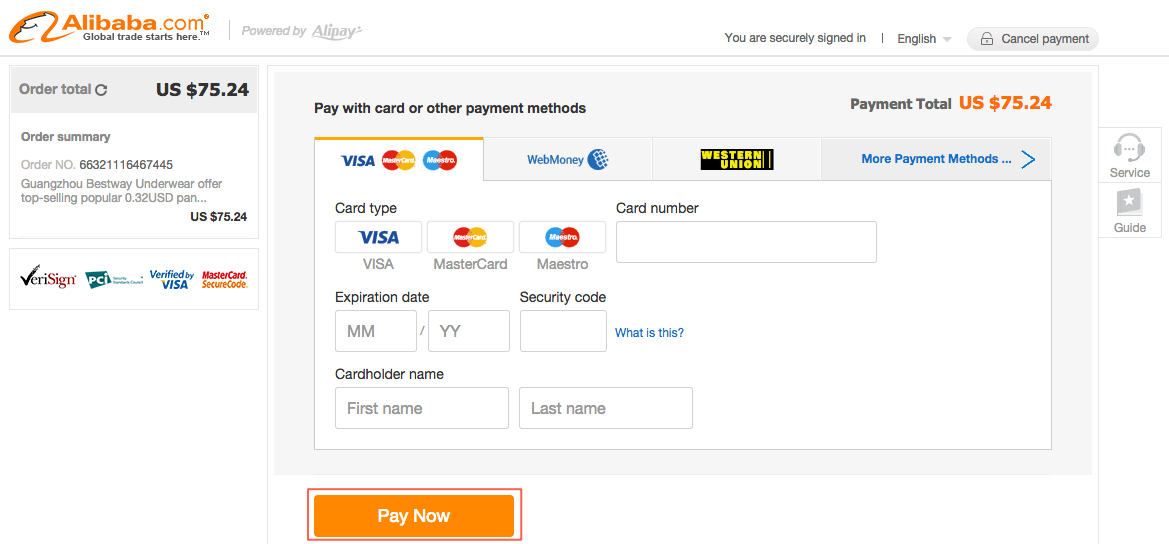The image showcases Alibaba.com's payment screen, prominently displaying the Alibaba logo and its tagline "Global trading starts here," with a "Powered by Alipay" note faded in gray beneath it. In the upper right corner, it indicates that the user is "securely signed in," with an English language option and a gray "Cancel Payment" button nearby. 

The left side of the screen features an "Order Total" box at the bottom, showing a total amount of "US $75.24" in bold, accompanied by an order summary and order number. 

Centrally positioned is the section for entering credit card information. A "Visa" option is highlighted, with alternative payment methods such as Web Money, Western Union, and more listed alongside it. The highlighted Visa option elaborates further, showing choices for Visa, MasterCard, and Maestro card types. Fields for the card type, expiration date, cardholder's name, and a prominent "Pay Now" button are clearly displayed, facilitating a seamless payment process.